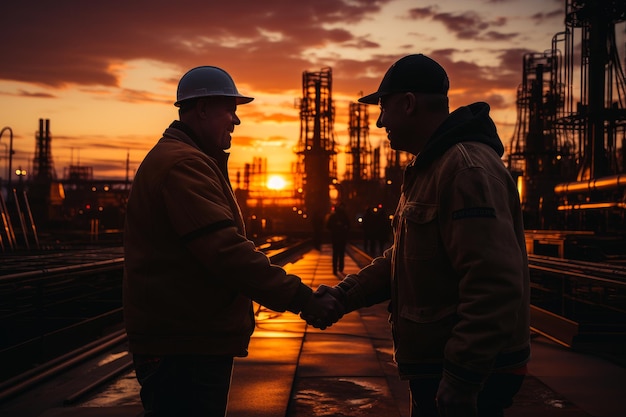The photograph captures a moment of two men shaking hands at what appears to be a construction site or an oil refinery during sunset. The man on the left wears a white hard hat and a brown jacket, likely with orange safety gear, while the man on the right sports a dark baseball cap and a similar heavy coat. The setting sun casts a stunning array of orange and purple hues across the sky, reflecting warmly on the slightly wet ground. Large metal machinery with pipes and poles define the industrial backdrop, as blurred refinery towers loom in the distance. Additional workers are scattered across the scene; one walks on the wet ground at the center, while two others move along what seems to be a street or railway. The overall ambiance suggests the end of a workday, framed by the breathtaking colors of a setting sun.